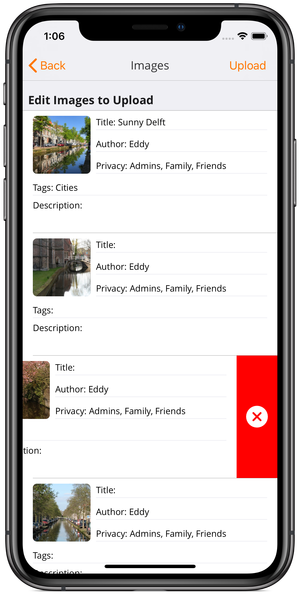A detailed close-up image of a cell phone screen displaying a photo management or editing application. At the top of the screen, the time reads 1:06, and the battery icon indicates it is nearly full. The interface shows an option to "edit images to upload," along with four image thumbnails in a list format.

1. The first image thumbnail is of a waterway with the title "Sunny Delft." The author is listed as Eddie (spelled E-D-D-Y). The privacy settings are marked as "admins, family, and friends," and the image is tagged under "cities." The description area for this image is blank.
   
2. The second image has an empty title field, is authored by Eddie, and shares the same privacy settings: "admins, family, and friends." Both the tags and description areas are blank.

3. The third image thumbnail is slightly cropped on the left side of the screen. It also lacks a title but lists Eddie as the author and has privacy settings of "admins, family, and friends." The tags and description fields are blank. Notably, this entry has a tall, skinny red rectangle with a white circle inside it featuring a red X on the right side.

4. The last image in the list has mostly blank fields except for the author's name, Eddie, and the privacy settings of "admins, family, and friends."